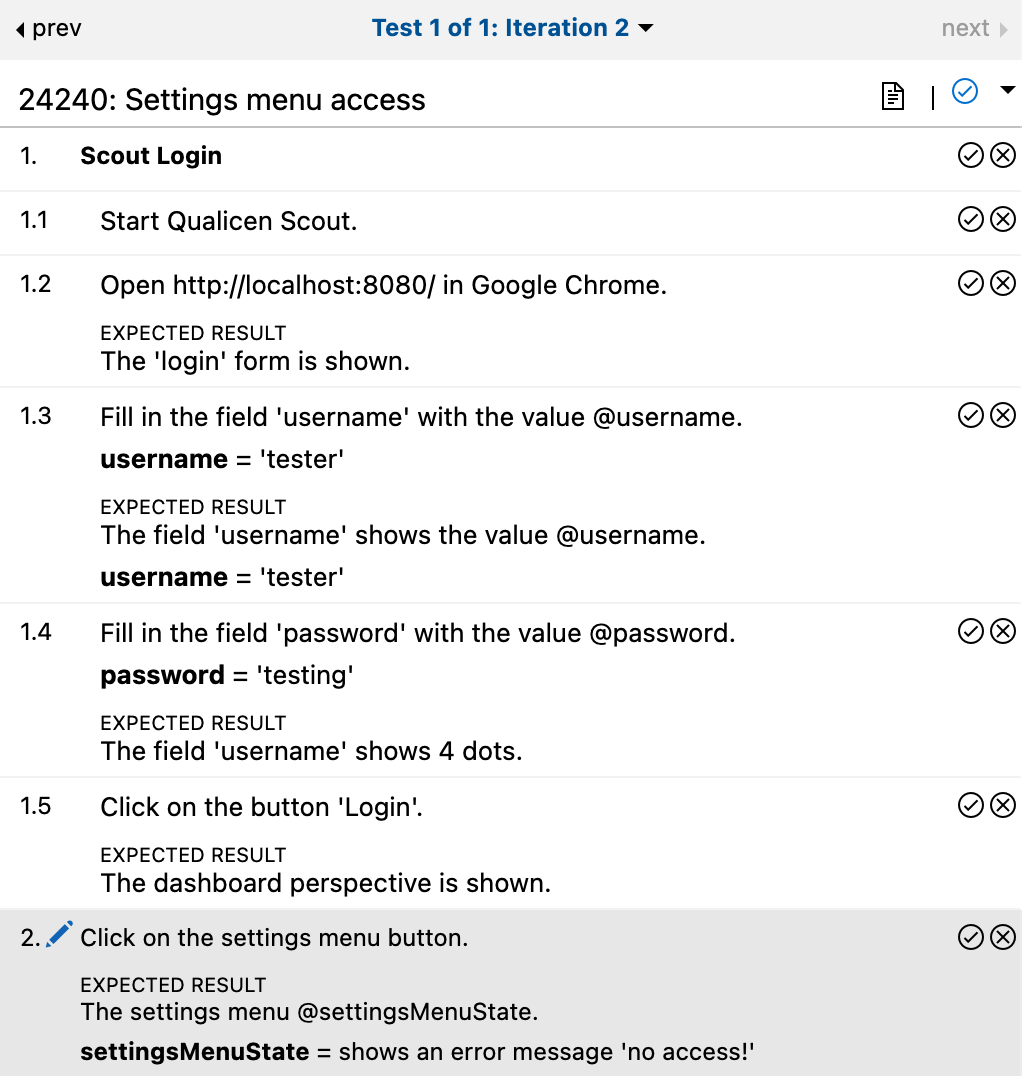The image depicts a detailed web page interface, particularly focusing on navigation and test process documentation. 

#### Top Navigation Bar:
- **Left Side:** A "Previous" button with a left-facing arrow labeled as "PREB."
- **Center:** The text "Test 1 of 1: Iteration 2" in blue, accompanied by a drop-down arrow.
- **Right Side:** A "Next" button with a right-facing arrow in light gray.

#### Secondary Navigation Line:
- **Elements:** The sequence "24, 24, 0: Settings, Menu, Access" followed by white space.
- **Icons:** An icon of a sheet of paper, a vertical line, and a blue circle with a blue X in the middle on a white background, accompanying a drop-down menu.

#### Step-by-Step Documentation:
1. **Scout Logon Process:**
   - **1.1 Start Call:** Send scout request.
   - **1.2 Open:** Navigate to the specified web page.
   - **1.3 Fill in Fields:**
     - Username.
     - Password.
   - **1.5 Click:** Press the "Login" button.
   - **Expected Result:** The dashboard perspective is displayed.

2. **Settings Menu Navigation:**
   - **Shaded Box (Step 2):** 
     - **Action:** Click on the settings menu button (depicted with a pencil icon).
     - **Expected Result:** The settings menu state should be updated.
   - **Bold Text:** "Settings menu state = chosen error message and no access!"

This caption provides a comprehensive and structured description of the web page's interface and the procedural steps outlined within it.